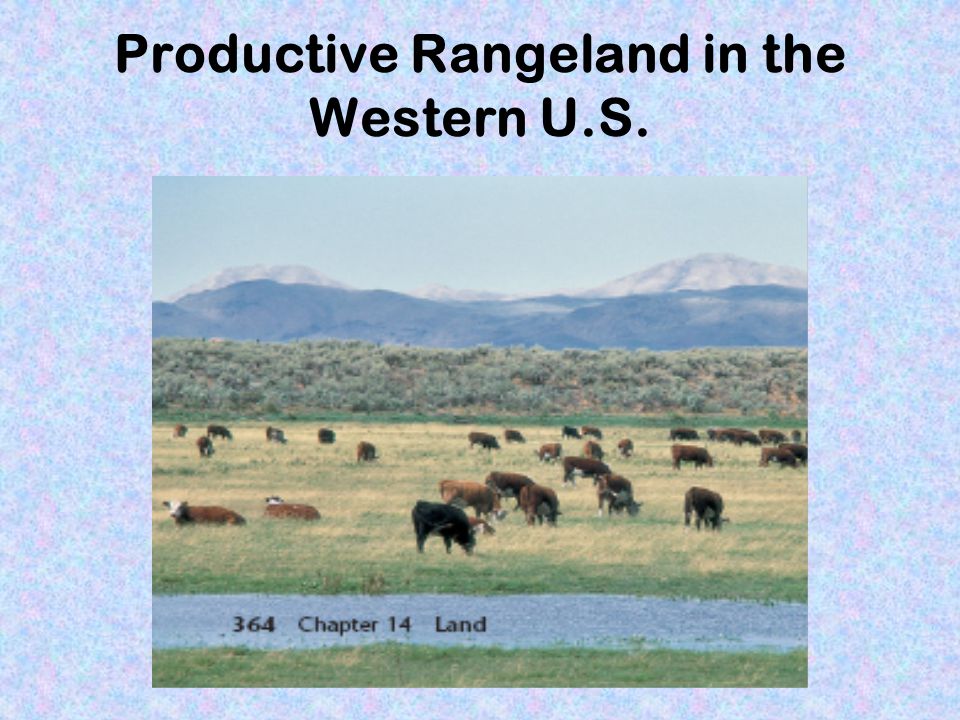The image features a speckled, marbled background composed of light purple, light pink, and light blue hues blending seamlessly together. At the top of the image, there's a black sans-serif caption that reads, "Productive Rangeland in the Western U.S." In the center, a scene depicts a tranquil mountain range with towering peaks transitioning from a dark gray to lighter gray as they recede into the distance. Below, the landscape unfolds into a grassy green hill, possibly an embankment of trees, leading to a lush, green-yellow mixed field sprawling across the frame. The field is dotted with cattle in various positions; some are grazing while others rest, showcasing a spectrum of colors including brown, black, light brown, and patches of white. A small stream meanders through the foreground, bordered by patches of grass. Adding to this picturesque scenery, a black text overlay near the water reads, "364 Chapter 14, Land." The entire scene is bordered by a static-like edge blending darker blue, lighter blue, and light purple tones, enhancing the image's overall aesthetic appeal. It is a bright, clear day, with the serene blue sky complemented by the distant mountain range.